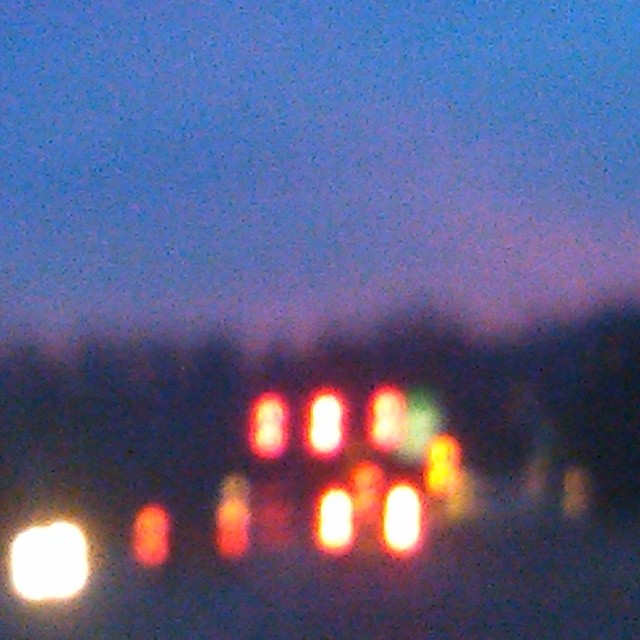This photograph, seemingly taken at twilight or shortly after dusk, captures a scene through an intensely blurred lens, reminiscent of the unfocused vision experienced without glasses. Dominated by a wash of indistinct red and white lights, likely emanating from car headlights, the image conveys an overwhelming sense of uncertainty and obscurity. The hazy landscape, punctuated by shadowy forms that could be distant trees, merges seamlessly into the darkening sky. Wisps of reddish clouds linger at the zenith, further hinting at the time of day. Overall, the photo is characterized by its extreme lack of clarity and focus, offering a dreamlike, almost disoriented view of nightfall on an indistinct road.